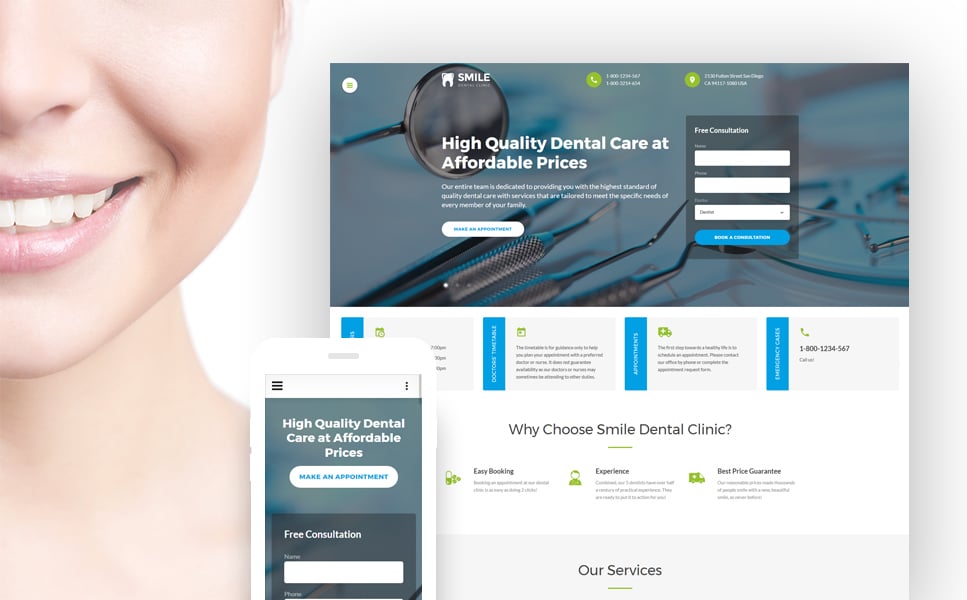The left side of the image features a close-up of a white woman. Her eyes are not visible, but her white cheek and half of her mouth are prominently shown, adorned with nude pale-colored lipstick. Her right white teeth are also slightly visible. 

The right side of the image displays a pop-up resembling a generic stock image on a white background, though the overall tone is darker. This includes silver dental instruments and a white tooth with the word "Smile" above it. Below "Smile" are details that are hard to make out, alongside a green circle containing a white phone icon, which seems to denote two different 1-800 numbers that are illegible due to small text size. There is also a circular icon with a GPS marker, which probably indicates an address that is similarly unreadable.

The leftmost section of the image contains the text, "High Quality Dental Care at Affordable Prices." Following this, there is a longer statement: "Our entire team is dedicated to providing you with the highest standard of quality dental care with services tailored to meet the specific needs of every member of your family." Below this text is a white button with blue text that reads, "Make an Appointment Now."

On the right-hand side, there's a gray box labeled "Free Consultation," with fields to write your name, phone number, and other details from a drop-down menu, but these fields are unreadable. Underneath the consultation box, blue text on a white background, gray text on black, or white text on gray background lists a 1-800 number to call and reasons why one should choose the Smile Dental Clinic.